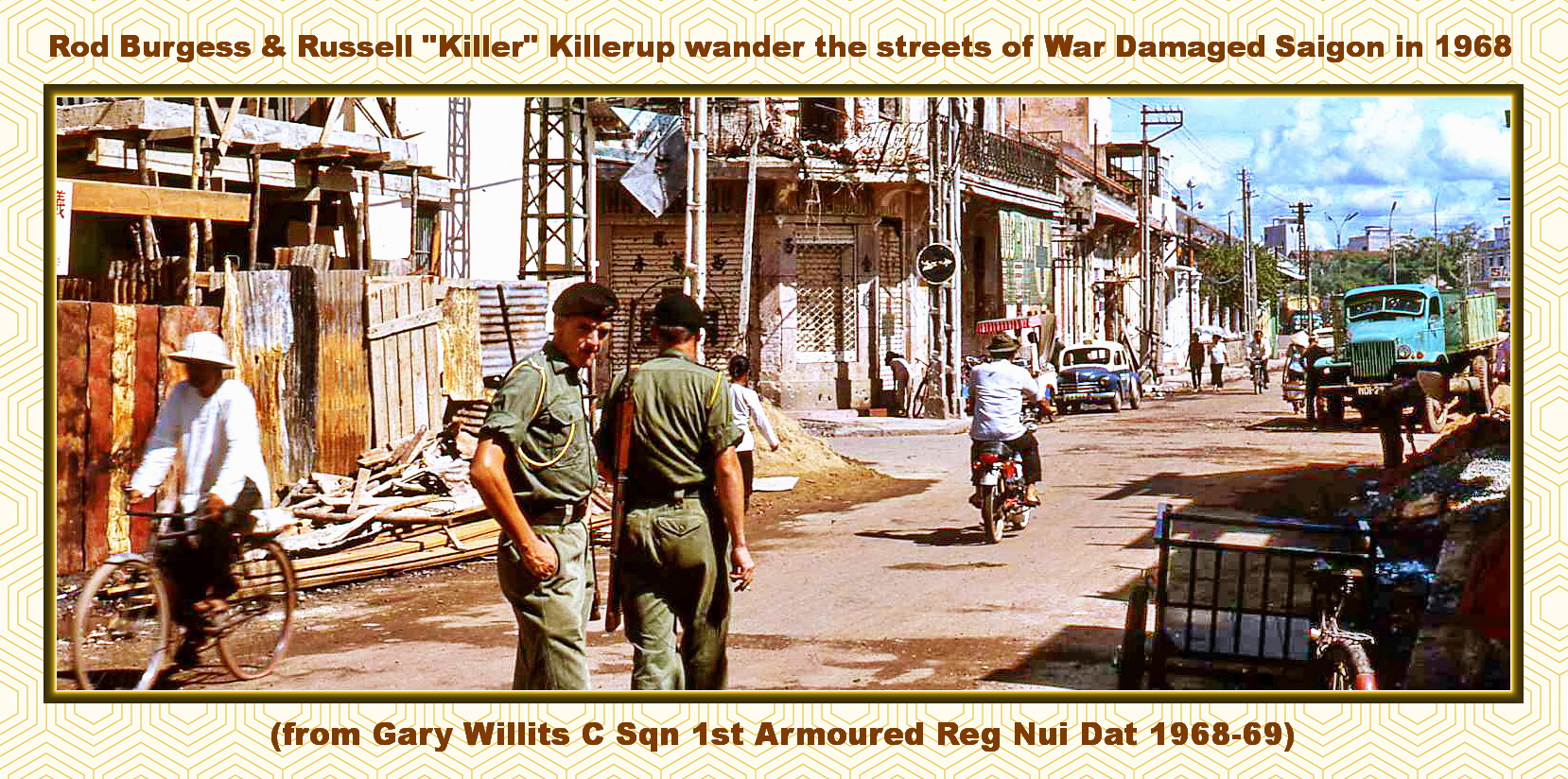This image is a colored photograph capturing a street scene from war-damaged Saigon in 1968. At the top, the text reads "Rod Burgess and Russell Killer Killerup wander the streets of war-damaged Saigon in 1968," while the bottom caption notes, "From Gary Willett's SQN, 1st Armored Regiment, Nui Dat, 1968-69." The photograph showcases two military personnel dressed in faded green uniforms and a blue hat, walking down a dirt street lined with decrepit and damaged wooden buildings. The street is strewn with wood debris and dirt, stretching into the distance under a bright blue sky. In the scene, there are also several civilians: a person on a bicycle to the left wearing a white hat and shirt, another individual on a motorcycle, and other people milling about. Visible in the background is a light blue truck and other cyclists, adding to the bustling, yet chaotic atmosphere of the war-torn street.